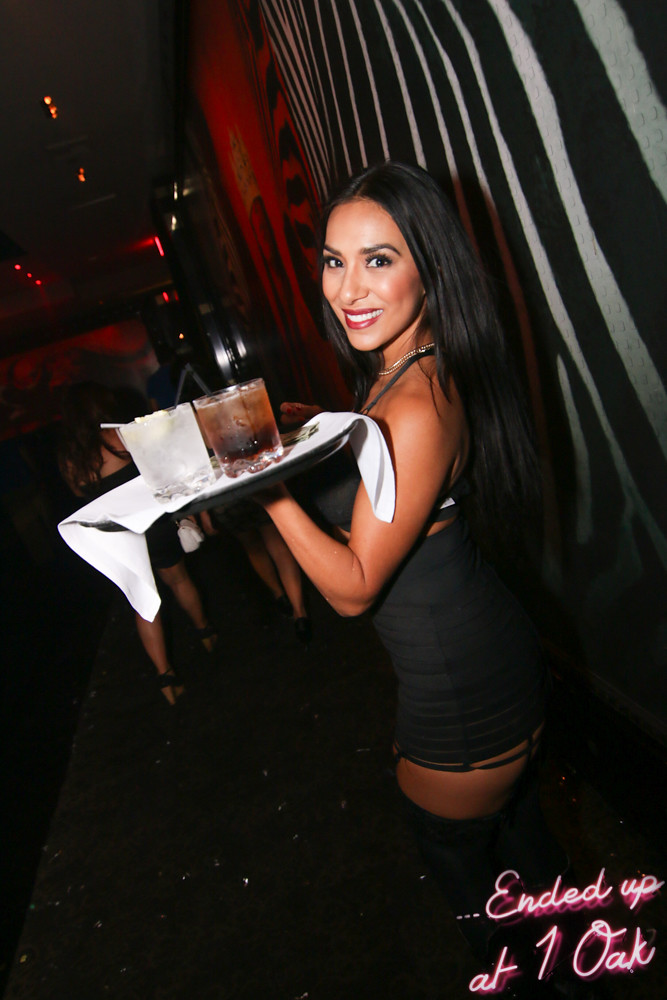In this dimly lit nightclub setting, a young woman stands center stage, capturing the viewer's attention. She has long black hair and is dressed in a sleeveless black mini dress, smiling directly at the camera. In her hands, she balances a tray covered with a white cloth, topped with drinks and ice, suggestive of her role as a server. The flooring is a dark carpet, setting a dramatic tone for the scene. More patrons can be seen to the left, adding to the bustling atmosphere of the club. The interior walls feature a mix of red with elaborate designs and black-and-white patterns, while the ceiling is adorned with sleek LED lights. In the background, subtle red lighting enhances the nightclub's vibrant yet intimate vibe. Notably, the bottom right corner of the image displays the text "Ended up at One Oak" in funky, disco-inspired fonts, grounding the setting firmly in its colorful, energetic environment.